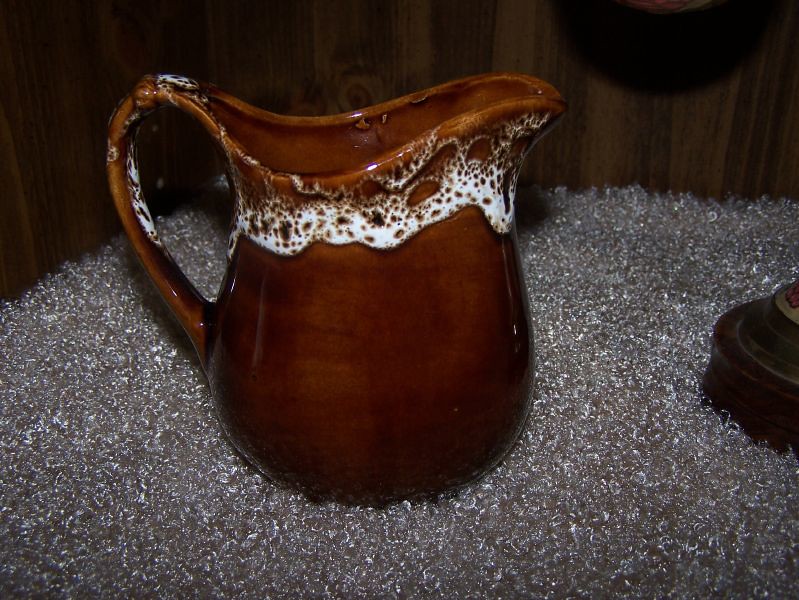The image showcases a dark brown drinking pitcher, possibly made of porcelain or ceramic, with a shiny, reflective surface that is somewhat matte yet with a sheen. The pitcher features a prominent handle on the left-hand side, designed with a high, contoured structure that creates a groove and culminates in a pointed top. The pitcher is intricately detailed with what appears to be a white, foamy pattern resembling bubbles or soapy water, especially concentrated around the upper part of the handle, extending across its front and sides. The setting includes a silvery-gray, plush polyester rug that serves as the backdrop, adding a tactile contrast to the smooth, lustrous finish of the pitcher.